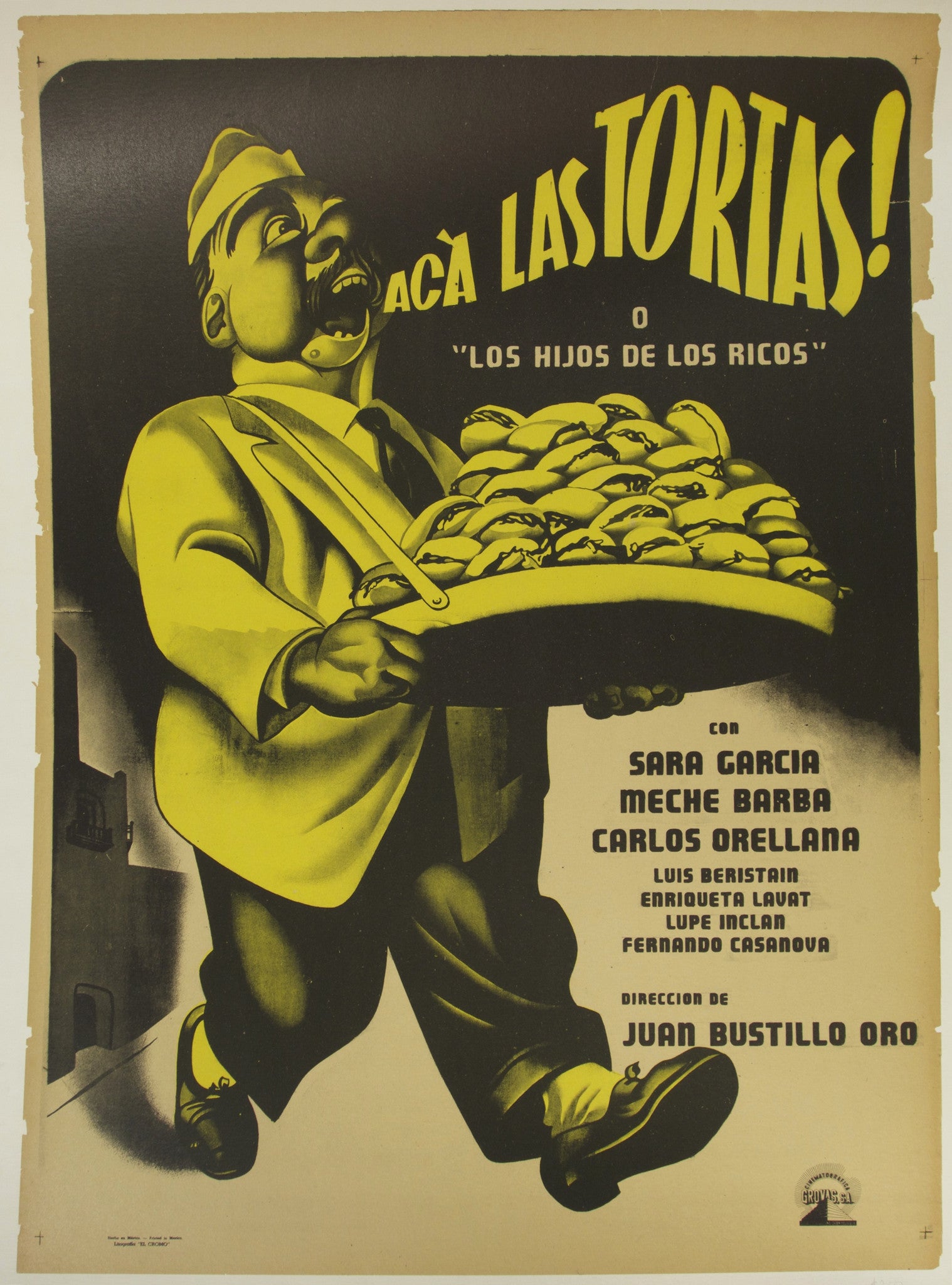The image depicts an old Hispanic movie poster with a faded beige background and black, greenish-yellow colors for the print. At the center is a cartoonish gentleman, portrayed as a waiter, wearing a white jacket suit, black pants, dark shoes, a tie, and a chef's hat. He has puffed-out cheeks and a mustache, and his open mouth displays Spanish text saying "Aca las Tortas" and "Los Hijos de los Ricos." He carries an old-fashioned shoulder strap tray laden with small buns or filled rolls, indicating his role as a server. The poster also features names of actors Sara Garcia, Meche Barba, and Carlos Orellana, along with the director Juan Bastillo Oro. This detailed and vibrant illustration suggests it advertises a vintage Hispanic film.